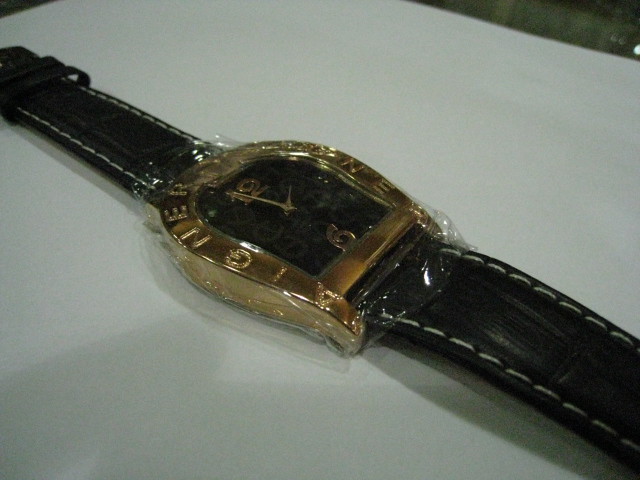This close-up photograph captures a wristwatch from a slightly angled overhead perspective, with the timepiece lying flat on a pristine white surface. The watch stretches diagonally from the bottom right to the top left of the image. The band, likely made of leather, is black with contrasting white stitching along its seams, adding a sophisticated touch.

The watch face stands out with its unique horseshoe shape, featuring an oval top and a squared bottom, edged in intricately carved gold. The brand name, AIGNER, is inscribed in gold on both the left and right sides of the gold trim surrounding the face. The face itself is black, creating a striking contrast against the gold. Positioned at the top of the face is a gold numeral 12, while a gold numeral 6 is at the bottom. The hands of the watch indicate a time just shy of 2 o'clock. This detailed and elegant presentation showcases the watch's refined design and luxurious craftsmanship.